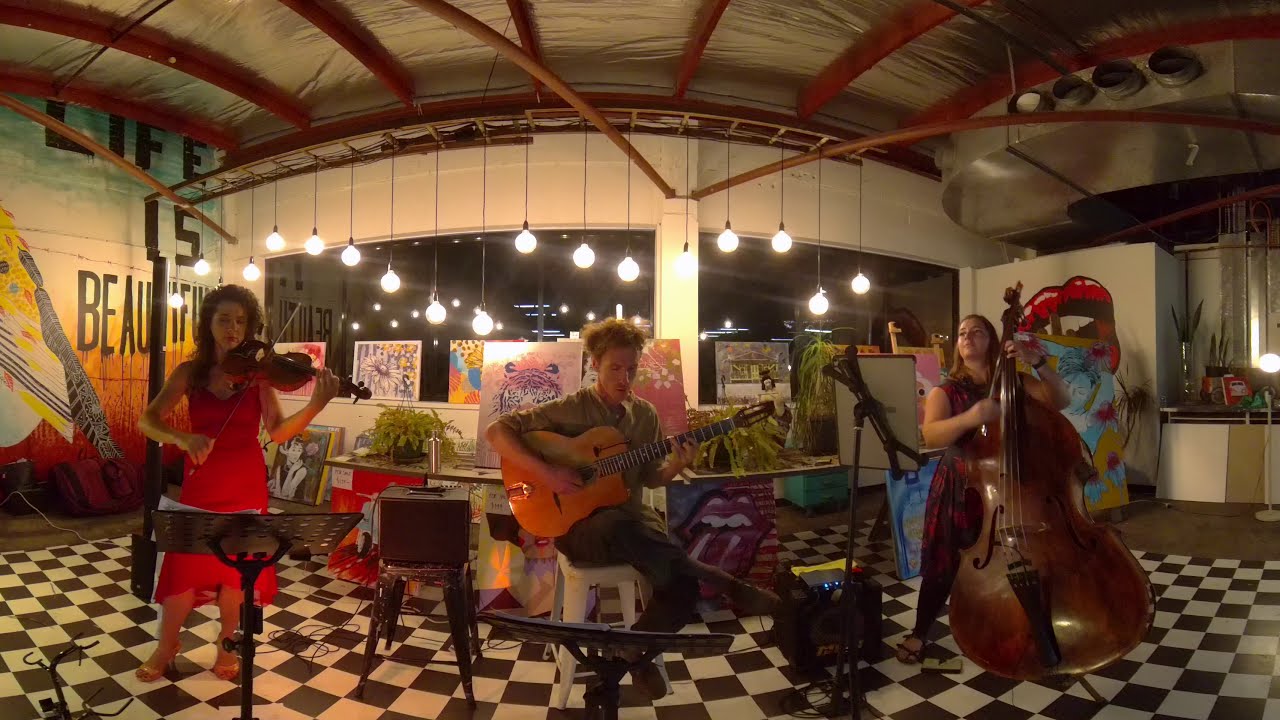The image showcases a dynamic trio of musicians performing in what appears to be a hybrid space that blends a cafe, art gallery, or small warehouse environment. The stage they occupy is set on a checkered black and white floor, contrasting against a backdrop filled with colorful murals, various paintings, potted plants, and globe lights hanging in a diagonal pattern from the ceiling.

In the center, a Caucasian man with short, slightly scruffy auburn hair and a long face strums an acoustic guitar while seated on a white stool. He dons an olive green shirt and brown pants, and his brown shoes rest casually crossed. To his left, a woman, also Caucasian with brown curly hair and red lipstick, is absorbed in her performance with a violin. She wears a striking red dress and has closed eyes indicating deep immersion in the music. A black metal music stand with holes in the frame is angled in front of her.

On his right, a woman in a long black and red floral dress stands tall, playing a stand-up bass. One of her hands blurs in mid-motion over the strings, capturing the energetic pulse of the moment. The other hand grips the neck of the bass. Her attire includes sandals, and her hair cascades in loose waves. The combination of the performers, the vivid backdrop, and the intimate setting creates a compelling snapshot of a rich, eclectic musical experience.

Behind them, the environment suggests a warehouse-like atmosphere with visible support beams and a mural that reads "Life is Beautiful," reinforcing the creative and artistic ambiance of the scene. The overall composition is visually rhythmic, echoing the harmony and vibrancy of the music being played.